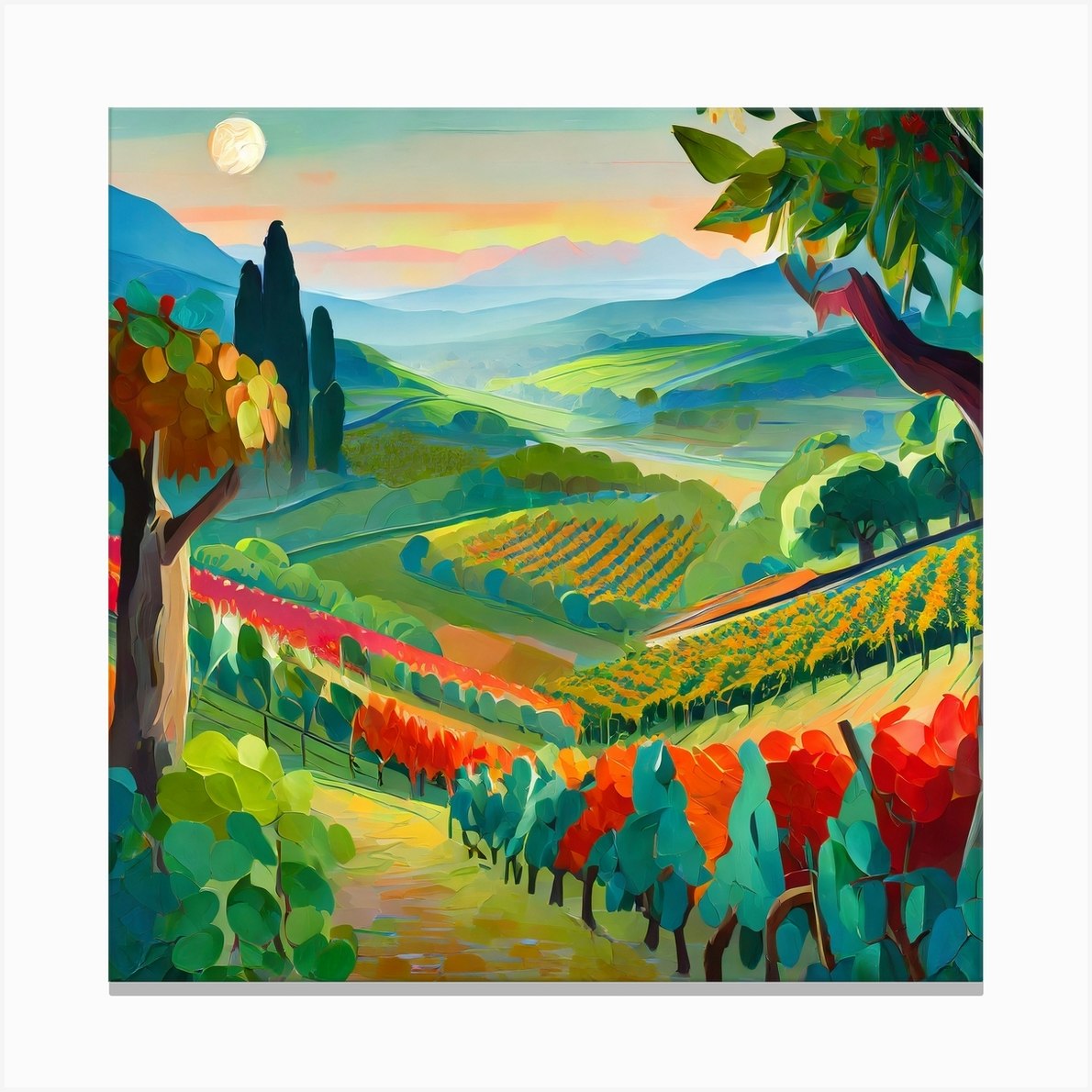This vibrant, watercolor painting, bordered by a thick white matte, showcases a picturesque rural landscape, possibly inspired by an Italian vineyard. The scene captures an expansive, verdant valley nestled between mountain ranges, depicted in a bright and impressionist style. Strips of color in the sky hint at a dramatic sunset, with a white sun situated in the upper left corner, illuminating the panorama.

In the foreground, meticulously cultivated rows of plants stretch across the valley floor. These are not grapevines but a blend of flaming red and green foliage, potentially roses or other flowering plants. The lush fields are interspersed with various types of trees, including tall, skinny green ones and a tree with multicolored leaves near a pathway flanked by vibrant flowers.

The landscape features numerous trees, including two noticeable ones—a small tree on the far left and another with red fruit or berries in the upper right corner. A rustic fence runs through the scene, and the overall palette is rich with warm tones of red, orange, yellow, green, and blue, adding to the impressionistic feel. The distant mountains and rolling hills provide a serene backdrop, completing this captivating depiction of a tranquil vineyard at sunset.